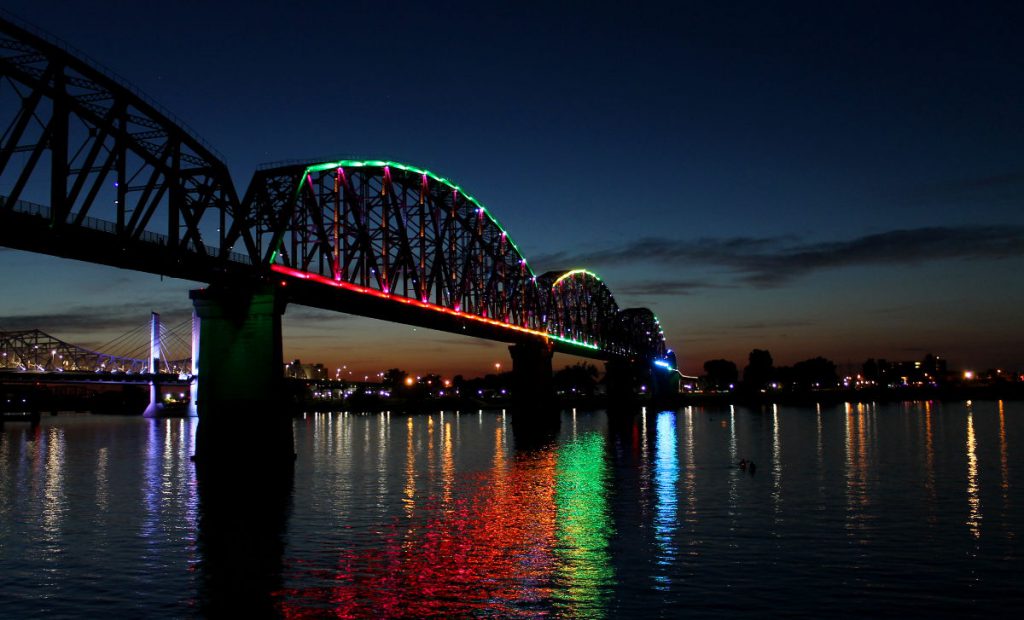The photograph captures a stunning nighttime view of a large and impressive bridge illuminated with Christmas lights. The bridge, which spans across a wide body of water, features sections that are brilliantly lit with red, green, and white lights. The vibrant colors cast a beautiful reflection on the water below, creating a bright and festive aura. In the background, the lights from the distant buildings and homes twinkle and cast small spheres of light on the water's surface, adding to the enchanting ambiance. The sky above is a deep, dark blue with occasional dark clouds, and near the horizon, hints of red and orange suggest the remnants of a recent sunset. The massive bridge is held up by giant cement pylons and is an architectural marvel of steel and light. To the left of the main bridge, a suspension bridge can also be seen, adding to the urban landscape that stretches towards the silhouetted city in the distance. The scene is dotted with stars, enhancing the nighttime atmosphere of this impressive cityscape.